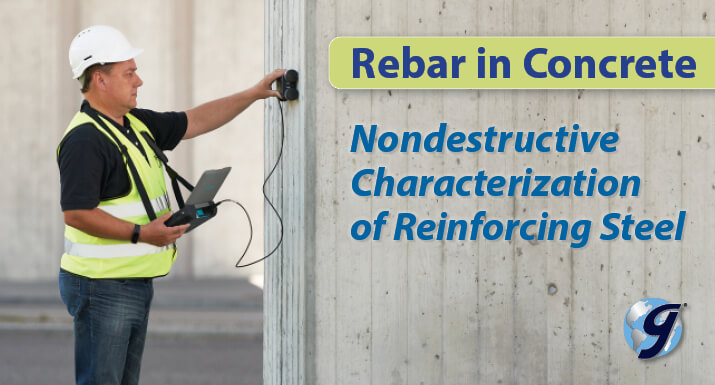The image is the title graphic for an informational booklet. It is a comprehensive color photograph featuring a man dressed in blue jeans, a yellow high-visibility (hi-vis) reflective vest, a white hard hat, and a black shirt. He is holding a small laptop computer with a black, square sensor attached via a cord. The man appears to be using the sensor to take measurements or readings against a wooden wall or concrete structure. To the right of the image, there is a prominent yellow rectangle with blue text that reads "Rebar and Concrete: Non-Destructive Characterization of Reinforcing Steel." Additionally, a logo displaying a stylized letter "G" over a depiction of planet Earth is located in the bottom right corner of the graphic.